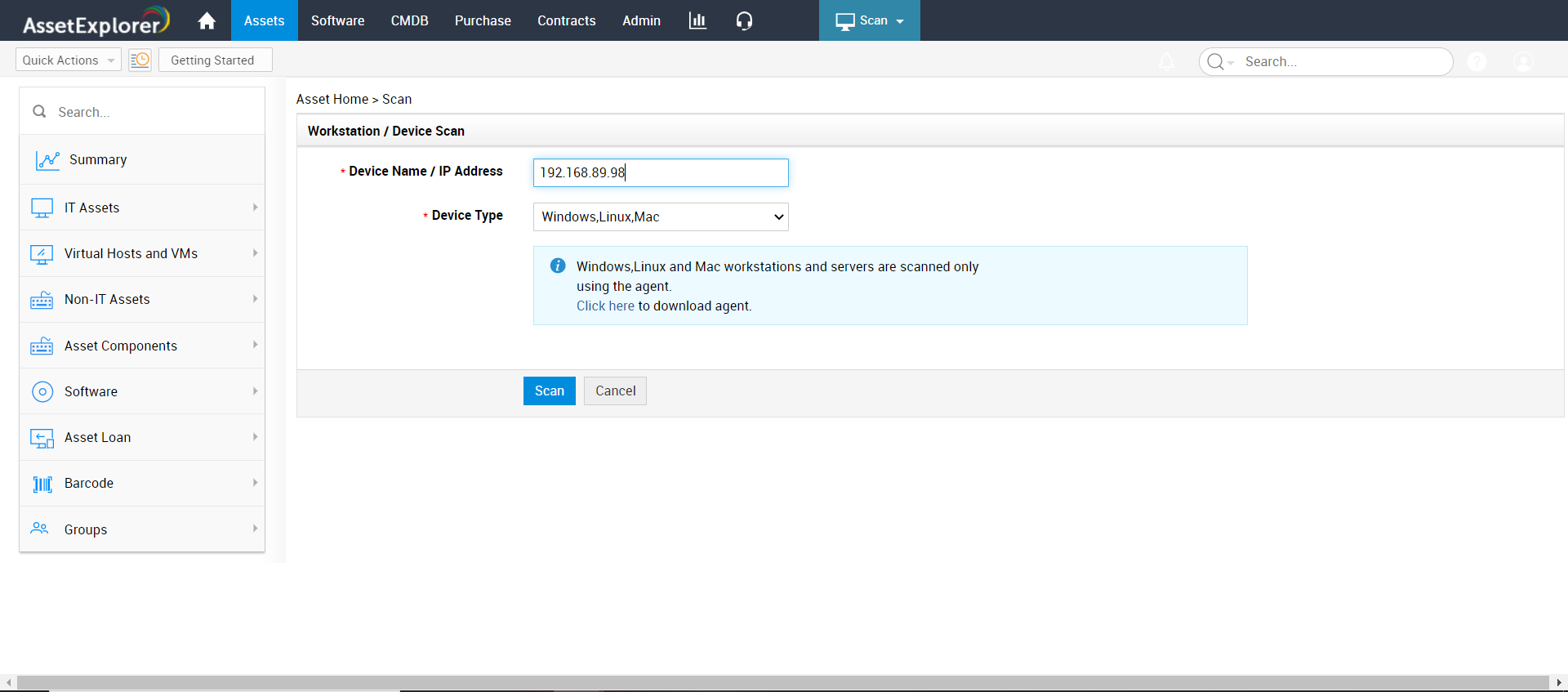The screenshot depicts a webpage from the "Asset Explorer" application. At the top left corner, the website's name, "Asset Explorer," is prominently displayed. Adjacent to it, a "Home" button is visible, followed by several navigation tabs labeled as "Assets," "Software," "CMD8," "Purchase," "Contracts," and "Admin." Additionally, there is a chart icon and a headphone icon. 

Below the navigation bar, the main section of the webpage is titled "Asset Home Scan." This section focuses on "Workstation/Device Scan," offering two input fields for user information. The first field is labeled "Device Name/IP Address," and the second one is labeled "Device Type." Beneath these fields, there is a conspicuous blue button labeled "Save." 

This detailed interface layout indicates that the webpage is designed for scanning and managing assets, particularly workstations and devices, within the "Asset Explorer" platform.